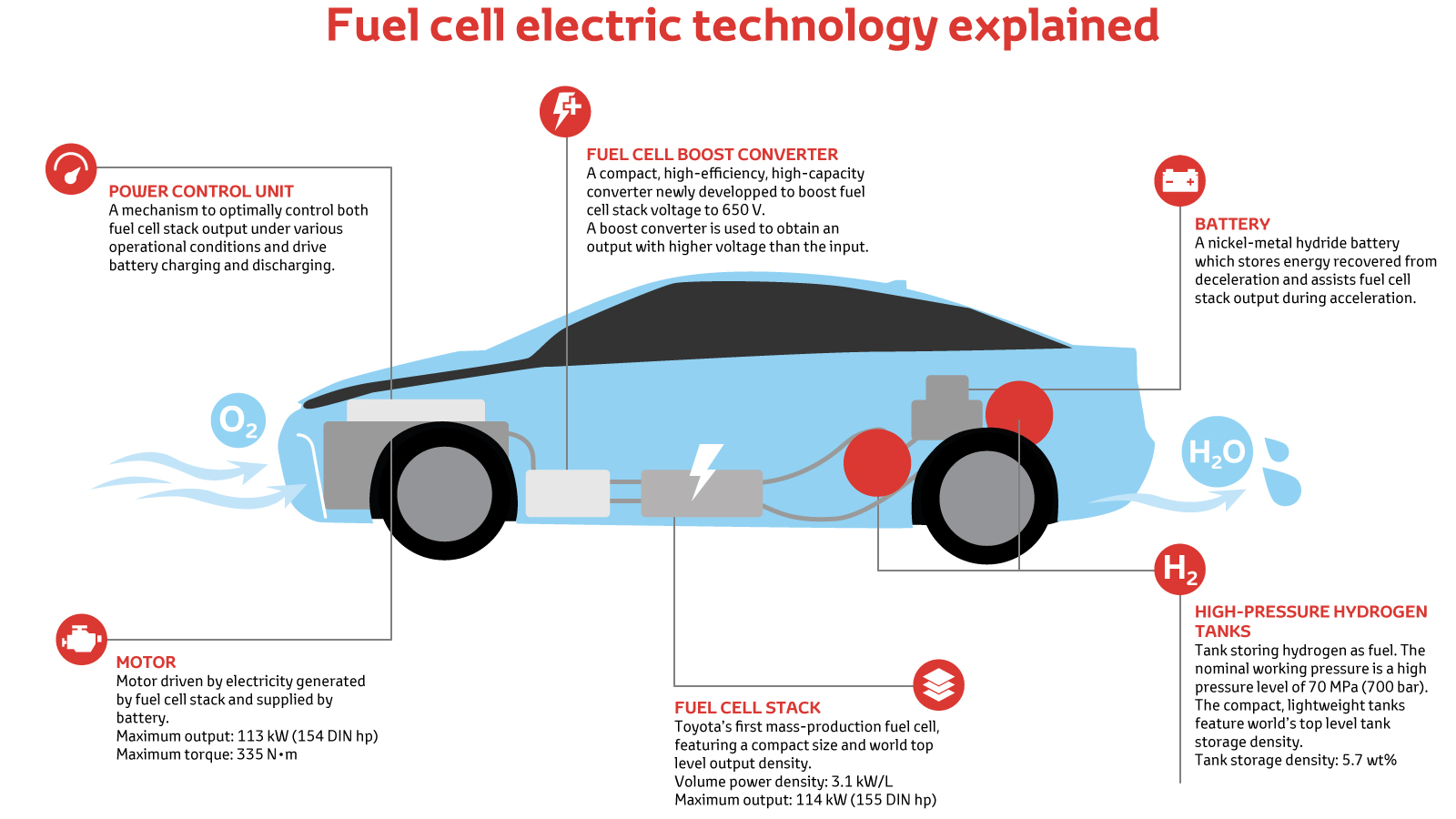The image is a detailed infographic drawing of a baby blue, cartoon-like car, viewed from the left-hand side. The car is set against a white background with no boundaries, and a red heading at the top reads, "Fuel Cell Electric Technology Explained," with only the 'F' in 'Fuel' capitalized. The car features a single elongated window that starts from the front and curves down towards the trunk, following the roofline.

Red circles, gray triangles, and a white lightning bolt mark various parts of the car, with lines connecting these symbols to six sections of explanatory text around the vehicle. Each section includes a red-encircled icon illustrating specific components: a battery, a fuel cell boost converter, a power control unit, motor, fuel cell stack, and high-pressure hydrogen tanks.

At the top front of the car, text explains the 'Power Control Unit,' followed by the 'Fuel Cell Boost Converter' in the middle, and the 'Battery' on the right. Each heading is in red, with smaller black text providing additional details. Icons above these text sections include a white battery, an abstract fuel cell boost converter, and a power control unit on a red background.

On the bottom left, the text 'Motor' is labeled with a red circle icon of a white motor, followed by 'Fuel Cell Stack' in the center with an icon showing a stack of white sheets, and 'High-Pressure Hydrogen Tanks' on the right, labeled with an H₂ symbol inside a red circle.

Additionally, a light blue circle with 'O₂' in white letters and black, curvy arrows represents oxygen intake at the car’s front. At the rear, another blue circle labeled 'H₂O' with white letters and accompanied by teardrop icons indicates water emission.

The overall design uses red and black lines to highlight the technological details of the car's fuel cell electric system.